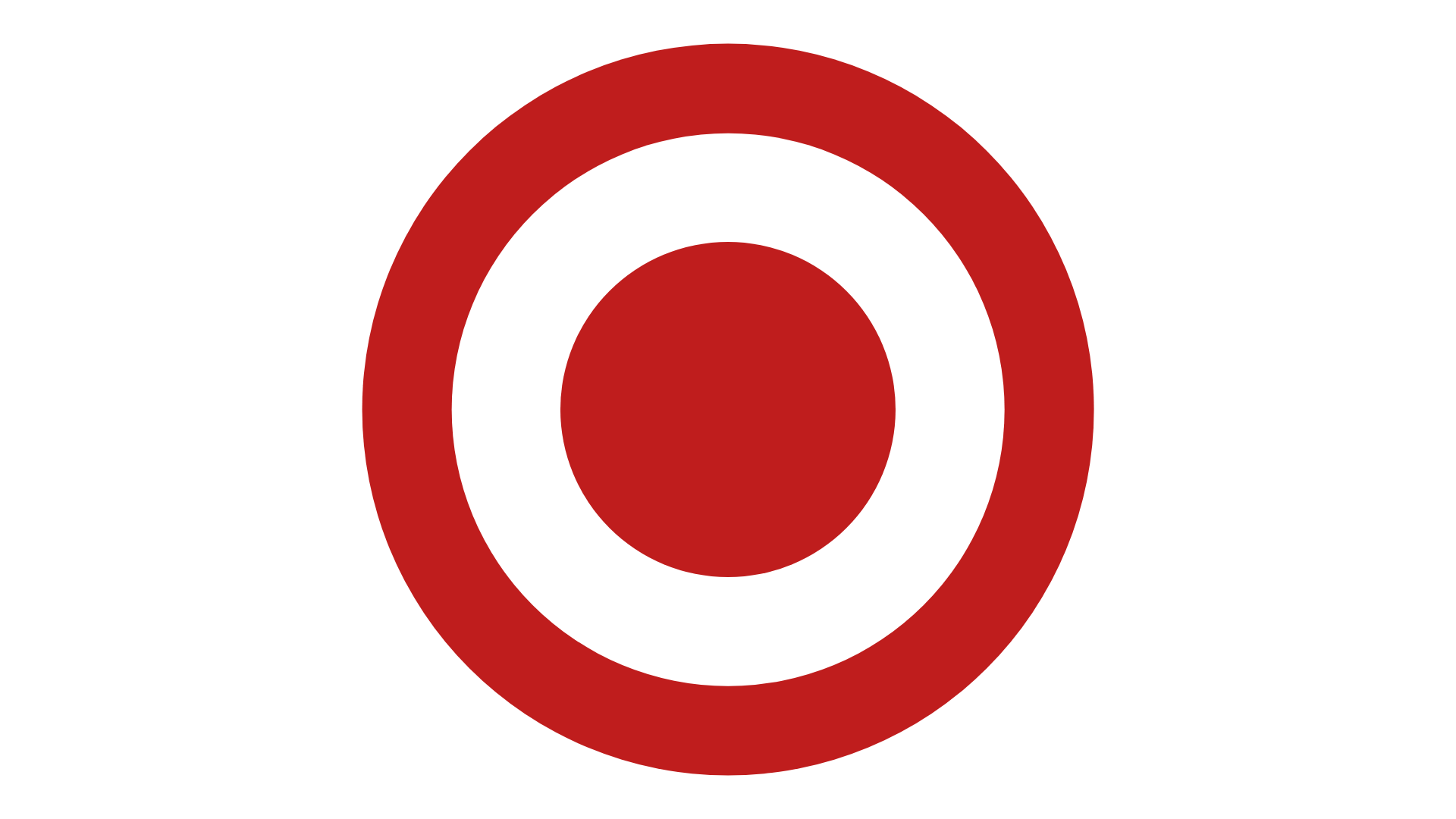This image depicts the Target logo, characterized by three concentric circles set against a pure white background. The outermost and innermost circles are dark red, while the middle circle is white, echoing a classic bullseye design. The image consists solely of these red and white elements, with no accompanying text, making it a simple yet distinct representation of the Target brand. The dark red inner circle, being the largest solid object, accentuates the iconic symbol’s central focus.